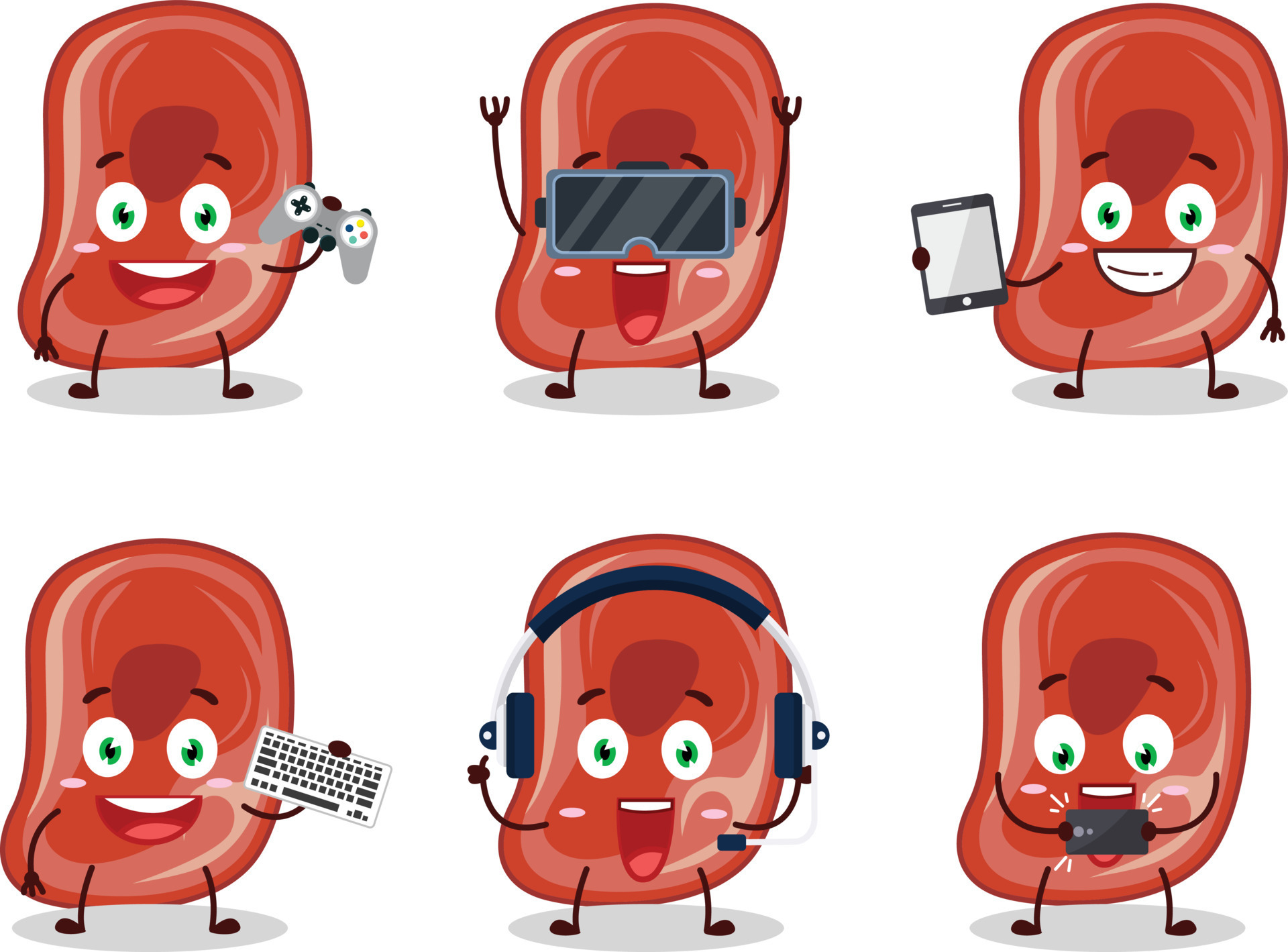The image features six cartoon depictions of a character resembling a red, steak-like figure with green eyes, stick arms, and legs that end in small, bulbous feet, each with three fingers. Arranged in two rows of three, each cartoon shows the character engaging with different pieces of technology. 

In the top left, the character is smiling broadly with raised eyebrows, holding a game controller in one hand. The top middle depiction shows the character with both hands raised, wearing VR goggles with its mouth open in excitement. The top right features the character with a toothy grin, holding a tablet in its right hand. 

On the bottom row, the bottom left drawing has the character smiling forward, holding a keyboard in its left hand. The bottom middle shows the character wearing a headset with a microphone, its mouth wide open and giving a thumbs up with one hand. The bottom right image shows the character looking down with an expression of concentration, holding a phone horizontally as if playing a game.